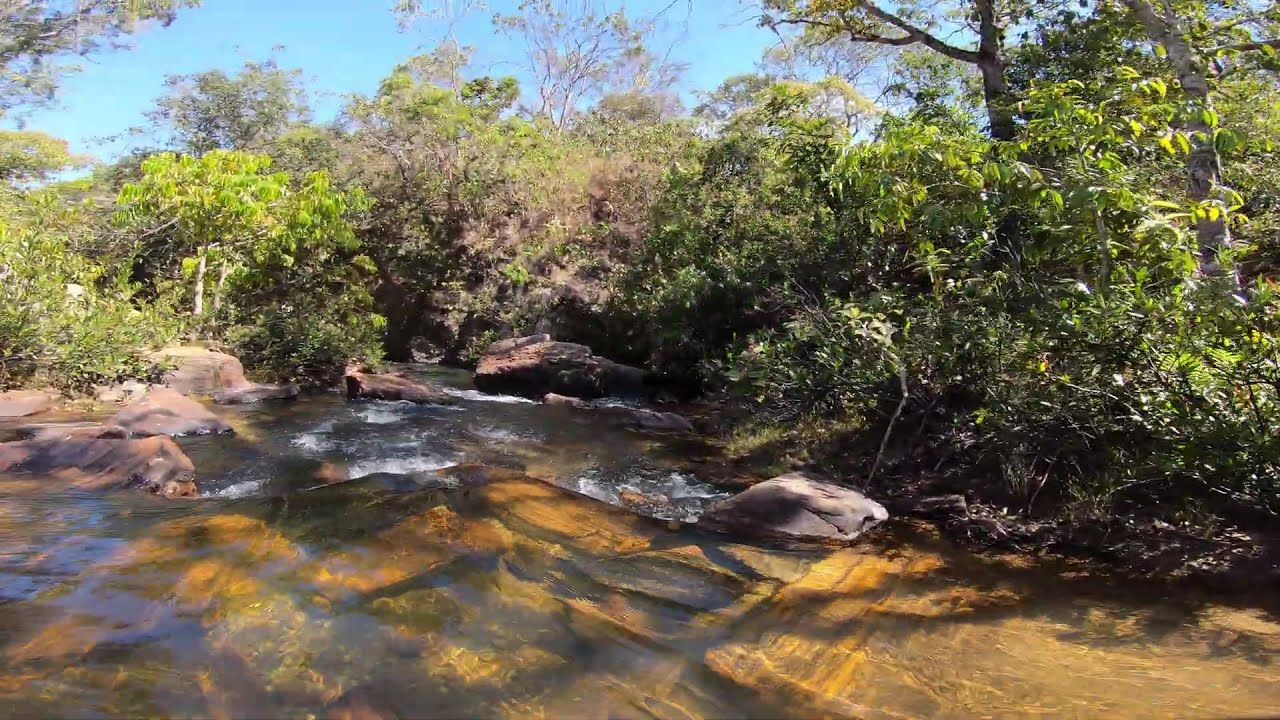This daytime photograph captures a serene outdoor scene featuring a shallow, narrow stream flowing through a natural, park-like setting. In the middle of the image, the stream, appearing crystal clear, reveals yellowish stones at the bottom, possibly tinted by sunlight. Large boulders, tinted brown, line both sides of the stream, with the water rushing over them, creating white, foamy pools as it cascades downstream. Surrounding the waterway, lush greenery thrives: tall trees and bushes dominate the landscape, though some trees exhibit a dry, brownish hue. Above, the sky is a brilliant turquoise blue, clear of any clouds, suggesting a sunny day. The overall tranquility of the scene is punctuated by the vibrant natural features and the dynamic movement of the water.